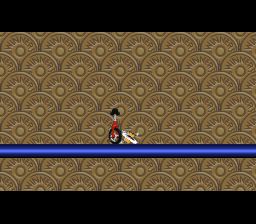The image depicts a piece of graphic art that appears to be a screenshot from a video game. At the top and bottom of the image, there are thin black borders framing the content. The central background features a series of golden, coin-like objects, each inscribed with the word "winner" and marked by a circular design in the middle, resembling the casing of a bullet. A prominent horizontal blue line stretches across the image about a third of the way up from the bottom. On this blue line, a unicycle with a black tire, black seat, and red frame is positioned. Adjacent to the unicycle, there is a yellow figure outlined with a white circle, seemingly depicting a person who has fallen off. This person appears to be lying on the ground, adding to the dynamic and somewhat whimsical nature of the scene.